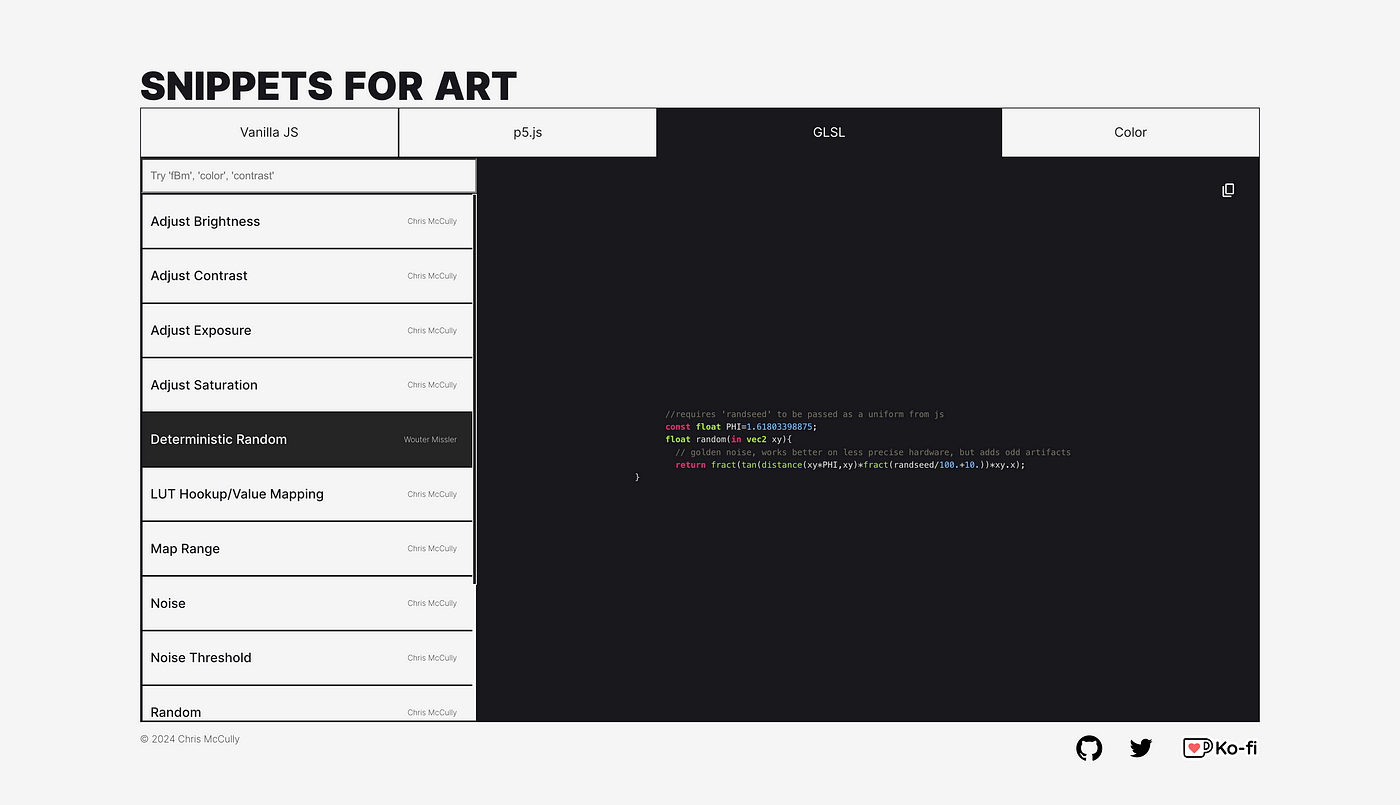The image showcases a screen capture from a digital platform, likely a webpage, associated with a software application called "Snippets for Art." It features a white background with the title "Snippets for Art" prominently displayed in capitalized bold black letters at the top left corner. Directly beneath the title, there are four tabs labeled "Vanilla JS," "P5.js," "GLSL," and "Color." The tab labeled "GLSL" opens up to a page with a predominantly black background displaying lines of code in various colors, including pink, green, and blue, although the text is too small to read clearly.

On the left-hand side of the screen, there are several horizontally listed categories, including "Adjust Brightness," "Adjust Contrast," "Adjust Exposure," "Adjust Saturation," "Deterministic Random," "LUT Hookup," "Forward Slash Value Mapping," "Map Range," "Noise," "Noise Threshold," and "Random." One of these categories is highlighted in black, making its title difficult to discern due to contrast issues.

At the bottom right corner of the image, along the white border, there are three icons: a headphone icon, a black Twitter (now known as X) icon, and a square icon featuring a red heart inside a white cup, which is identified as the Ko-Fi logo. The entire interface gives the impression of an online tool designed for artistic and coding adjustments, likely intended for editing or enhancing art projects.